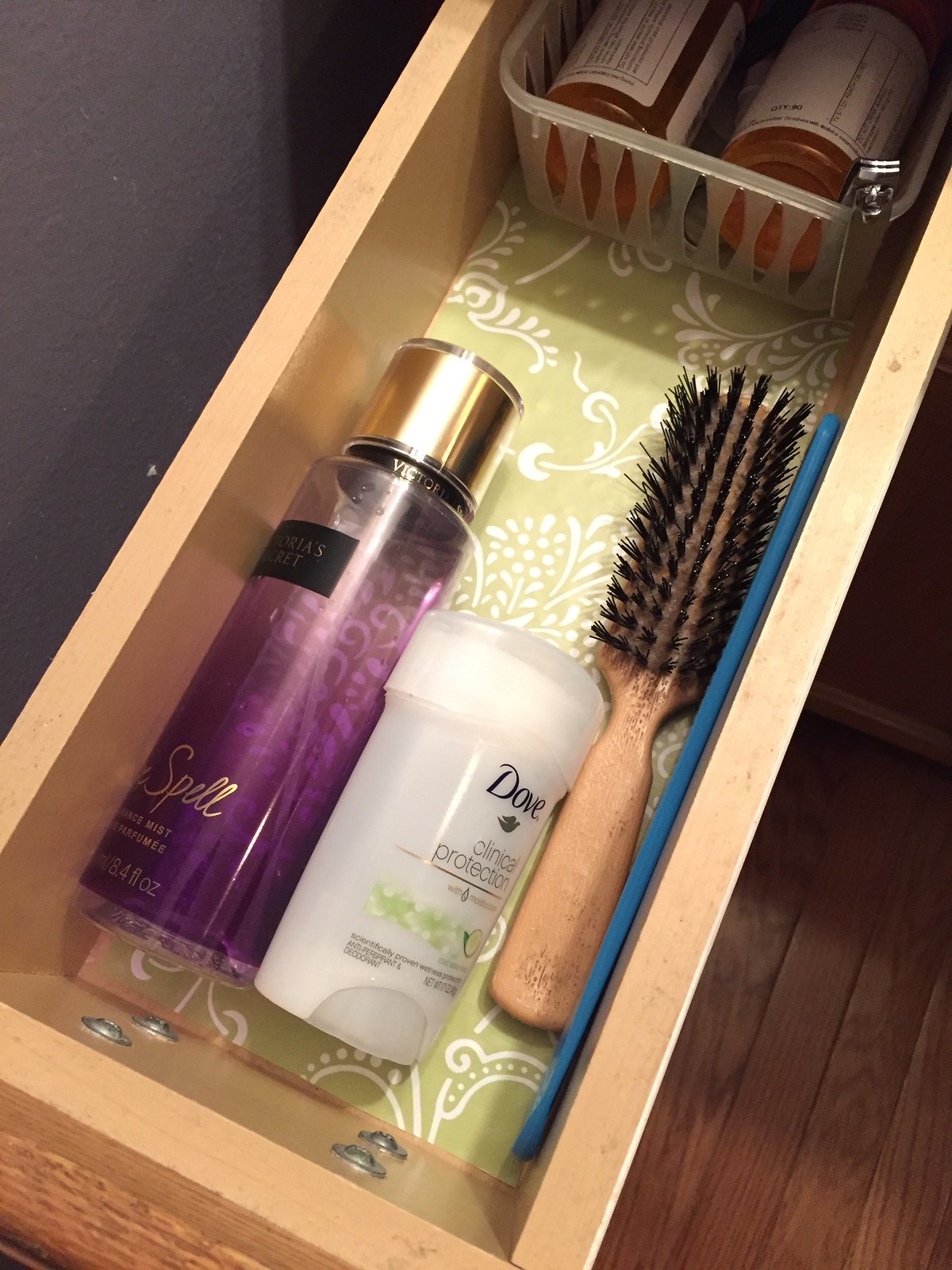The image showcases a collection of diverse items neatly arranged in a drawer or shelf. At the top, a transparent basket holds several orange prescription pill bottles adorned with white labels, accompanied by a nail clipper neatly perched on the edge. Below this, a bottle of Victoria's Secret perfume stands out with its clear container, gold cap, and alluring purple liquid inside. Adjacent to the perfume is a stick of Dove Clinical Protection deodorant. Nearby, a wooden brush with black bristles lies next to a mysterious long blue object. The base of this organizational space is adorned with a green liner featuring a delicate white leaf pattern. The surrounding environment reveals purple-painted walls and elegant hardwood floors, adding a touch of sophistication to the setting.